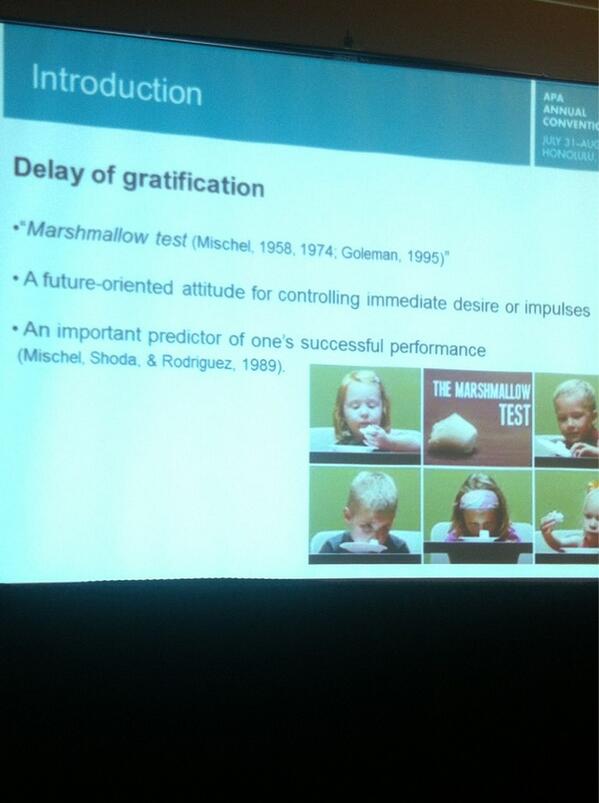The image is a photograph of a projected PowerPoint slide, likely taken during a presentation at the APA Annual Convention held from July 31st to August in Honolulu. The projection screen is the main visible element in the dark room, with no people, stage, or ceiling visible. The slide has a blue banner at the top stating "Introduction," followed by the text "Delay of Gratification." Underneath, several bullet points read: "The Marshmallow Test, Mischel 1958-1974, Goldman 1995," "A future-oriented attitude for controlling immediate desires or impulses," and "An important predictor of one's successful performance, Mischel, Shoda, and Rodriguez 1989." To the right of this text, there is a grid of images showing children interacting with marshmallows—some are picking up the marshmallow, sniffing it, or simply staring at it. The top middle image within the grid features the text "The Marshmallow Test" over a close-up of a marshmallow on a wooden surface. The slide visually reinforces the concept of delay of gratification through the famous Marshmallow Test experiment.